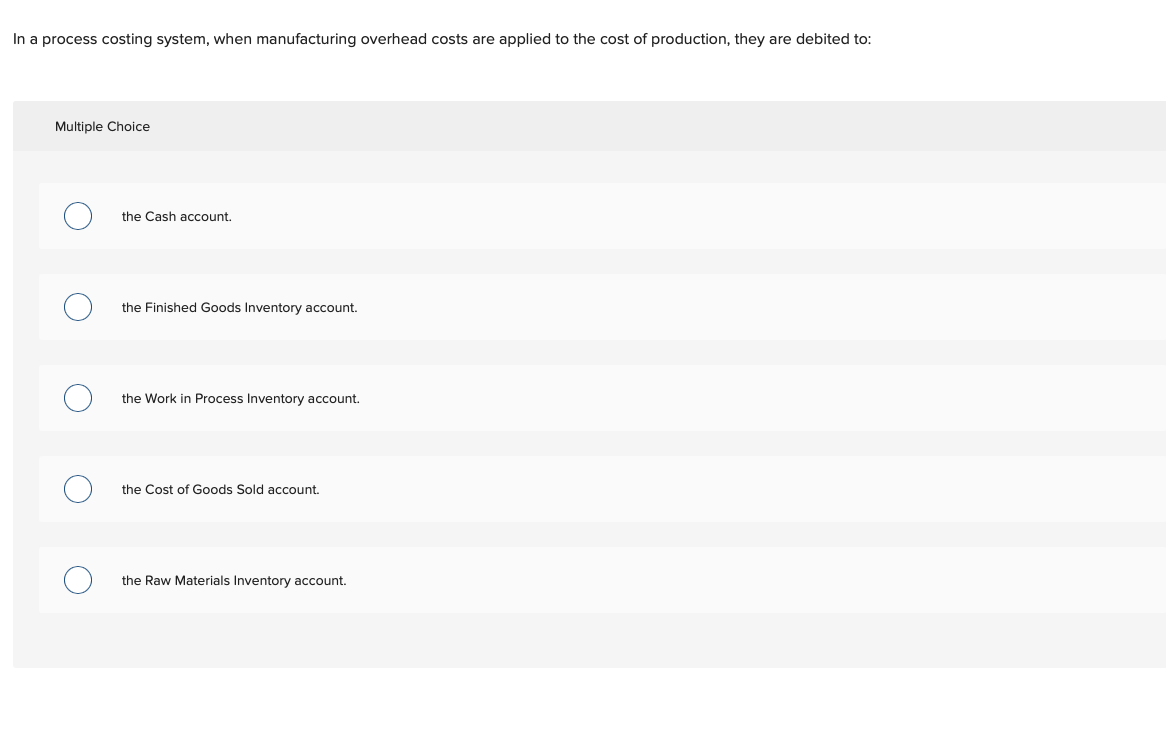This screenshot displays an interface for an online test or quiz, potentially related to an educational course or business training program. The interface is minimalist, featuring a clean and open design with little clutter. 

At the top of the screen, the test question is prominently displayed in clear text: "In a process costing system, when manufacturing overhead costs are applied to the cost of production, they are debited to:" Below this question, the answer format is stated as "Multiple Choice" on a subtly colored strip, which appears to be either pale gray or light beige.

Beneath this strip, five sizable radio buttons, depicted as empty circles, are lined up vertically as selectable options. None of the options are checked. The choices provided are as follows:
1. The cash account
2. The finished goods inventory account
3. The work in process inventory account
4. The cost of goods sold account
5. The raw materials inventory account

Currently, there is no visible button to proceed to the next question or submit the answer. It's possible that such a button only appears after a selection is made. Overall, the interface is straightforward and user-friendly, focusing strictly on the task at hand without any extraneous elements.